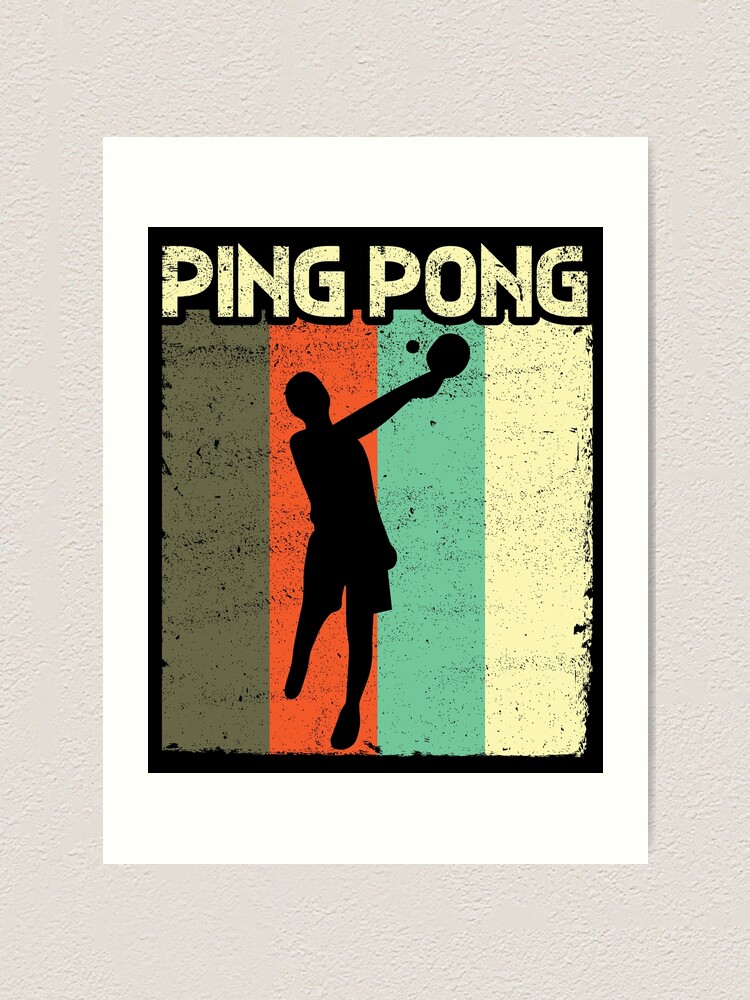The image is a poster displayed on a rough, white wall. The poster, which could also be mistaken for a t-shirt design or a computer-generated image, features a central silhouette of a person executing a wide swing in ping pong. This black silhouette contrasts sharply against four vertical stripes of color that serve as the background: a tone akin to a light brown with a greenish hue, a red or clay color, a teal or sky blue shade, and a yellow that matches the text of the title. The title "Ping Pong," written in a rugged, large beige or yellow font, appears prominently at the top of the image. This weathered and artistic design stands out on the white-bordered poster, creating an eye-catching centerpiece on the rough, white wall.